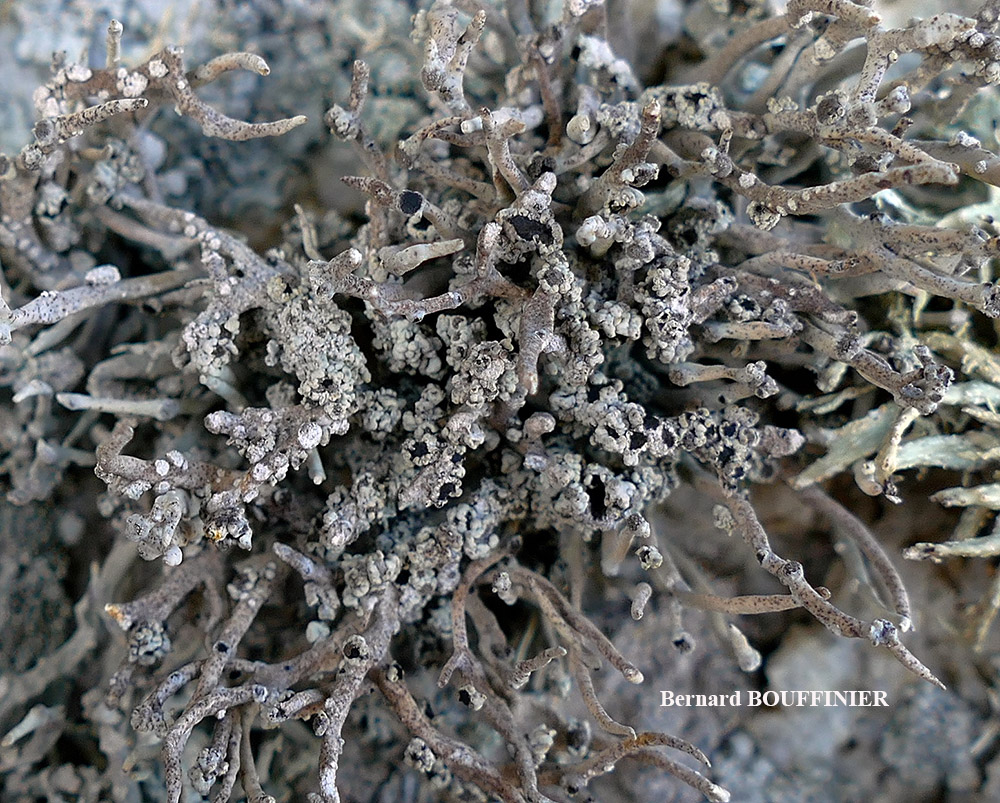This detailed close-up image captures a dense cluster of branch-like structures with a grayish-brown hue, possibly resembling either tree branches with fungus or coral underwater. The branches extend in various squiggly, organic directions, their tips adorned with small, gray chunks that have black tips, likely indicating some form of fungal growth. The background of the image is blurred and features more branches, contributing to the scene's complexity and organic nature. In the lower left corner, the name "Bernard Bouffanier," with "Bernard" in white and "BOUFFANIER" in all caps, is clearly printed. The lower right corner, slightly obscured and blurry, appears to reveal brown rocks underneath. The image overall manifests a palette of grays, whites, and browns, with a hint of lime green on some strands, adding a subtle touch of color to the otherwise muted scene.